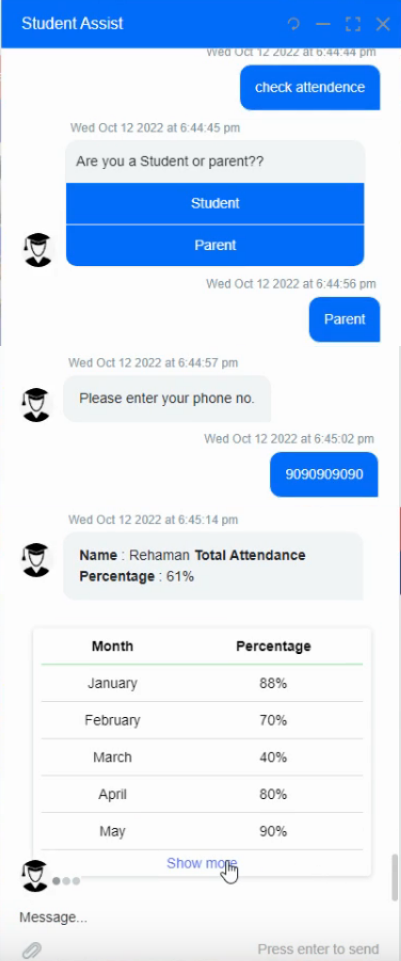This image is a screenshot from the "Student Assist" application. The interface features a primarily white background with key sections highlighted in darker blue. At the very top of the screen, a dark blue banner displays the title "Student Assist" in white text. Directly below, a blue rectangle contains the white text "Check Attendance," followed by the date and time: "Wednesday, October 12, 2022 at 6:44 PM."

The interface then poses the question, “Are you a student or parent?” against a dark blue background with white text options labeled "Student" and "Parent," accompanied by an icon of a student in a graduation cap with a blank white face. Immediately to the right of this, a blue button with the label "Parent" in white text is provided. 

Further down the page, the form instructs to "Please enter your phone number," which is filled into another blue box with white text. Below this section, various attendance statistics for a student named Rahman are displayed in a tabular format. Rahman's total attendance percentage is listed as 61%, with monthly percentages detailed as follows: January - 88%, February - 70%, March - 40%, April - 80%, and May - 90%.

At the bottom of the screenshot, the text "Show More" appears in blue, accompanied by a small hand icon pointing to this option, indicating it is interactive.